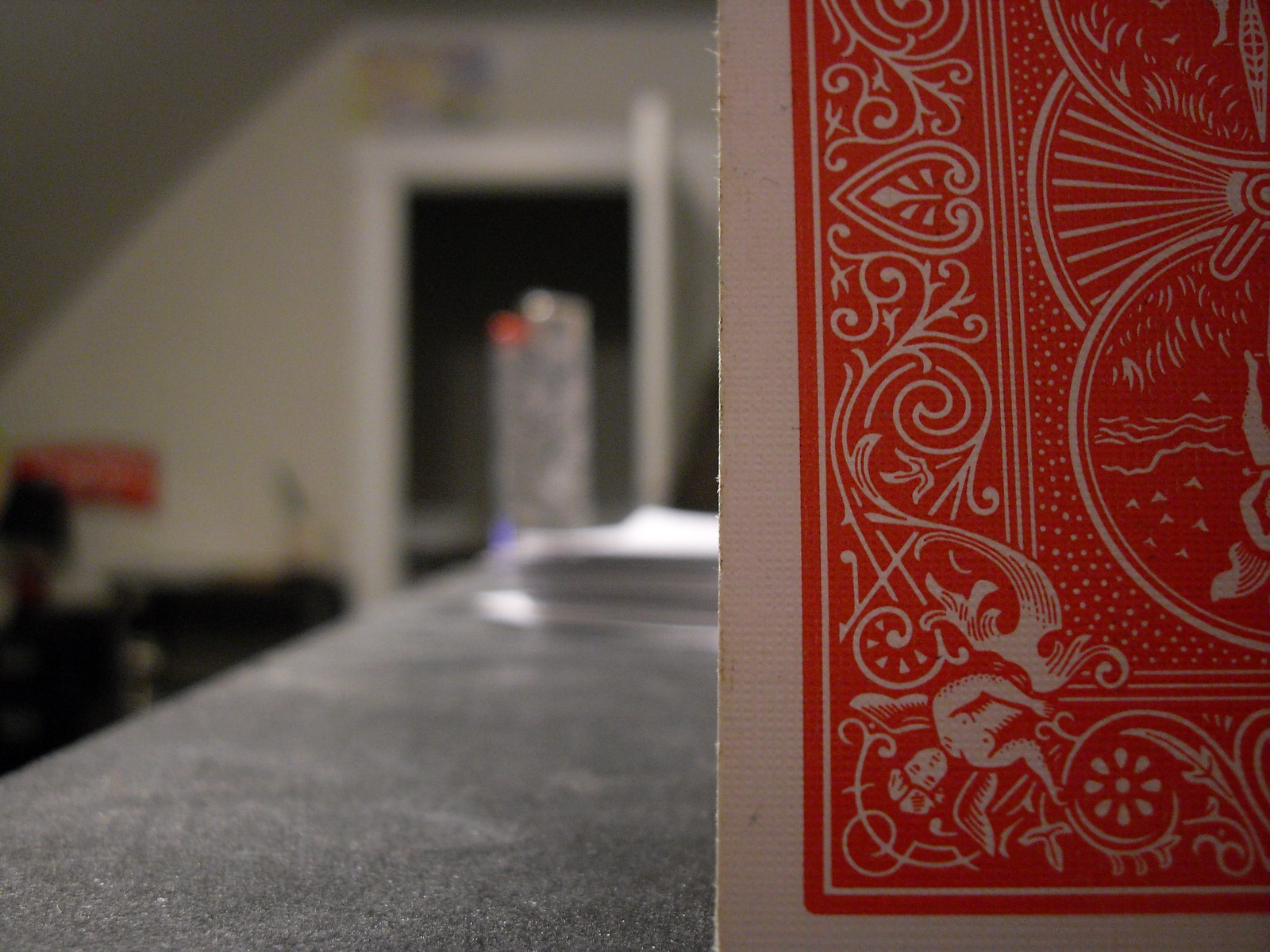The image depicts an interior room with light beige walls and an open white door, complete with a matching white door frame. In the background, there is a large, illuminated figure that appears somewhat ethereal due to the surrounding light. Above the door, a blurry sign in yellow and black is visible.

On the left wall, a small red sign is discernible, alongside a plant in a decorative floor vase. The room's floor is covered with brownish carpet that features a floral pattern. Scattered on the floor are various unidentified items.

A table with a gray tabletop holds a stack of papers and a striking playing card. The playing card is predominantly red with white edges, adorned with small white angels and large red circles. Part of a girl's body is also visible near the card. Additionally, a large black fan can be seen, along with red hearts interspersed with red and white elements throughout the scene.